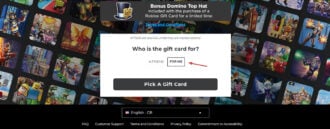The image depicts a cluttered, labyrinthine scene as though viewed from within a security monitoring room, but instead of security feeds, numerous television screens are displaying still images from various video games. The main focus of the image is a promotional element for a virtual item, with the prominently featured text "Bonus Domino Top Hat." Beneath this, the words "Who is this gift card for?" invite the viewer to select a gift card, accompanied by a black button. A red arrow is strategically placed, pointing towards a nearby white button, possibly labeled with instructions such as "Start Here" or "Pick Me." At the bottom of the screen, there is a black background area containing generic icons typical of user interfaces that likely offer options for language selection and additional information sections like "About Us." The overall purpose of the platform remains ambiguous, but it clearly involves video games and in-app purchase opportunities, centering around the acquisition of a virtual top hat accessory.